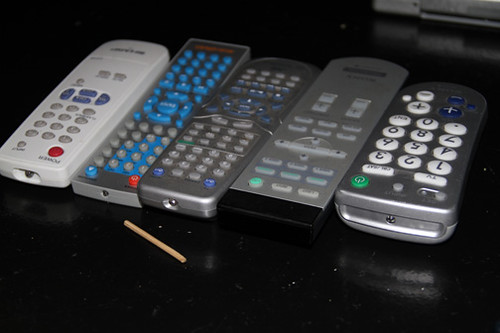This photograph captures a lineup of five remote controls positioned side by side on a glossy black tabletop. The remotes are facing the camera, allowing a view of their buttons and sensors. In front of the central remote rests an unlit matchstick, possibly missing its head. All the remotes are rectangular, with slight variations in size and shape. From left to right, the first remote is white with a multitude of gray and blue buttons, including a red power button. The second remote is silver or light gray and features gray and blue buttons, also with a red power button. The third remote follows the same color scheme with gray and blue buttons but lacks a distinct power button color. The fourth remote is silver with fewer buttons and a noticeable black border near the top, with a green power button. The fifth and final remote is silver with larger white and blue buttons, and a green power button. The shiny black surface beneath the remotes reflects their shapes and includes some white specks scattered across it, as well as a hard-to-identify gray device in the upper right corner, potentially a DVD player. The remotes appear to be well-used, given the variety of button layouts, suggesting they might belong to different devices or brands.